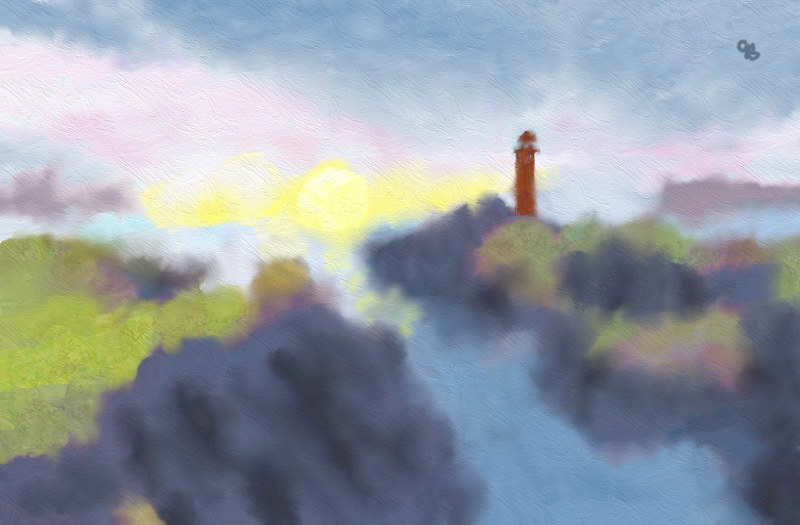The image is a detailed painting, likely utilizing watercolors or oil paints, depicting a serene sunset scene. The sky is a captivating blend of blue and pink hues, marked by a yellow sun that sits just above the horizon, casting a soft glow with rays extending outward. Central to the composition is a small, red lighthouse, positioned slightly to the right of center and higher up, subtly emerging from the hazy backdrop. The painting’s texture appears intentionally blurry, reminiscent of the dabbing method and further enhancing its tranquil ambiance.

In the foreground, to the bottom left, a patch of green represents grass and foliage atop cliffs or rocky terrain. This green area gives way to a body of water, whose deep blue tones suggest a bay or river winding toward the ocean. From the bottom right, a strip of dark, purplish land extends diagonally toward the center, interspersed with hints of vegetation. Another sliver of land is visible in the distant right background, completing the landscape.

Soft, fluffy clouds scatter across the sky, with a particularly vivid collection tinged pink near the sun. The overall effect of the painting is one of quiet natural beauty, achieved through a combination of flowing colors and slightly rippled textures that evoke the essence of watercolors or oil painting techniques.